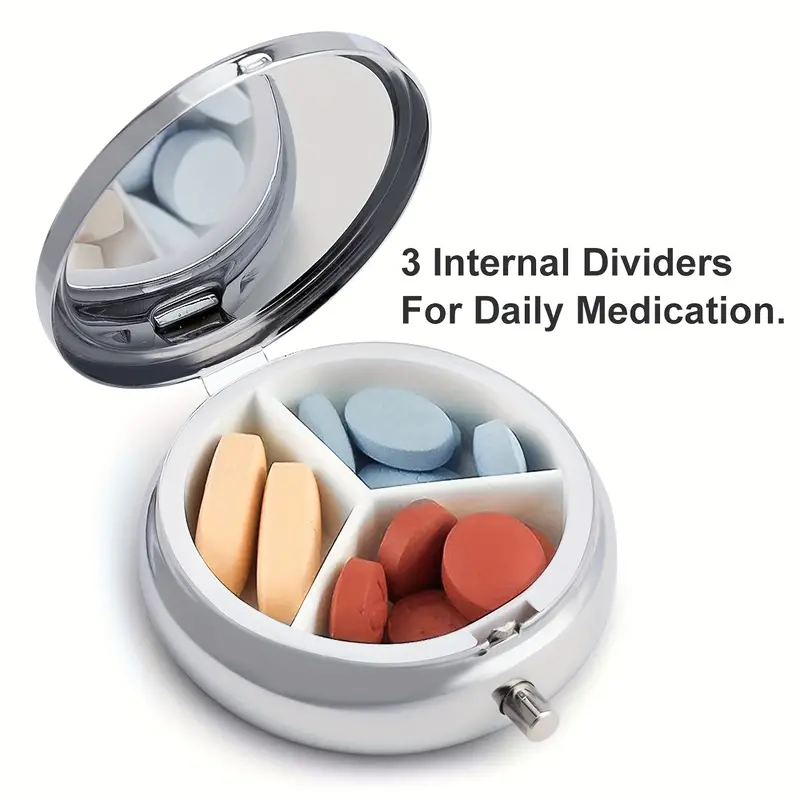The image depicts a small, round pill organizer designed for daily medication, set against a white background. The container, resembling a makeup compact or small disc, has a hinged chrome lid that opens to reveal a mirror inside. The interior is divided into three triangular compartments, arranged in a Y shape, each holding different colored pills: two yellow vitamins in the top left, several pale blue vitamins in the top right, and a group of red tablets at the bottom. Beside the organizer, in black font, is a caption that reads "three internal dividers for daily medication." The sleek design includes a simple switch to open and secure the lid, making it an ideal portable solution for organizing medications.